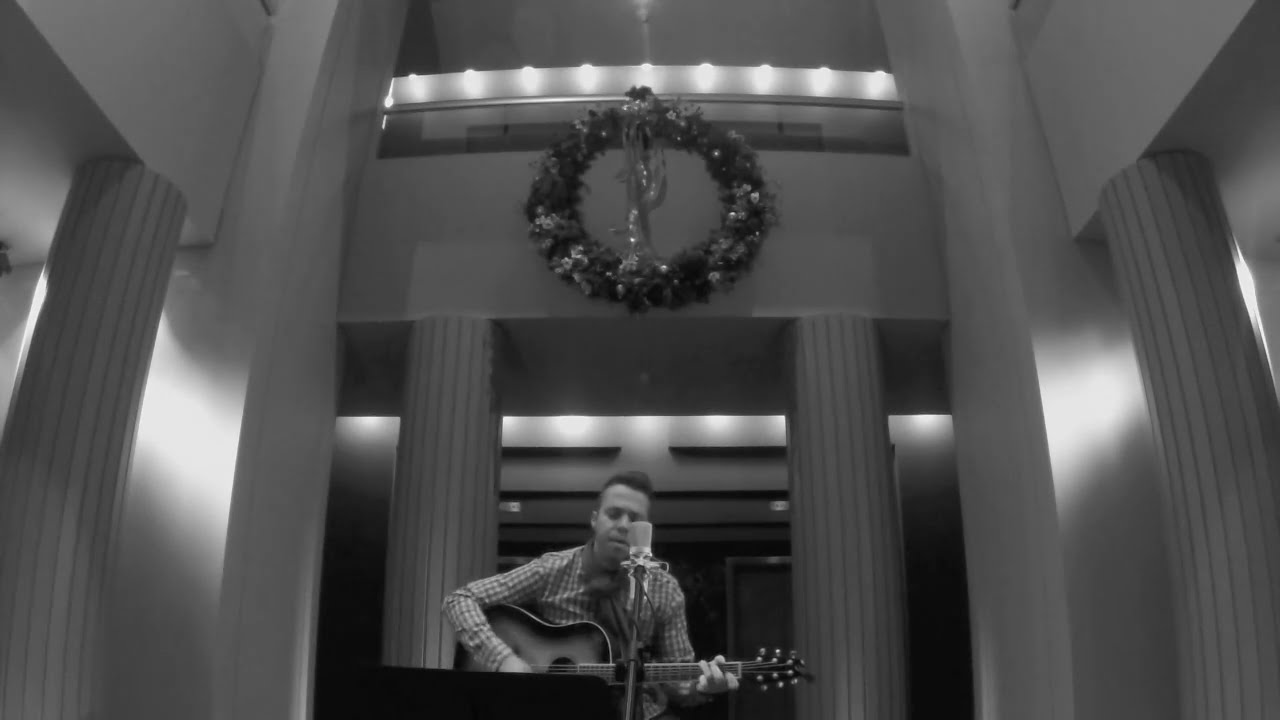In this black and white photograph, a man is positioned at the center, appearing to be in his mid-30s, with short hair styled upwards. He sits (or possibly stands) playing an acoustic guitar, wearing a plaid, long-sleeved button-up shirt with a collar. In front of him is a microphone on a stand, suggesting he is singing, even though his mouth is closed at the moment the photo is taken.

The room is grand and expansive with a high ceiling, supported by four tall columns—two on either side of him. Behind him, slightly to the right, there's a door. Above him, mounted on what appears to be a balcony structure, is a large, round Christmas wreath decorated with an assortment of festive elements, including what seems to be an angel in the center. The scene is well-lit, enhancing the detailed interplay of light and shadows characteristic of black and white photography. Although the audience isn't visible in the shot, it's implied that he is performing for a crowd.